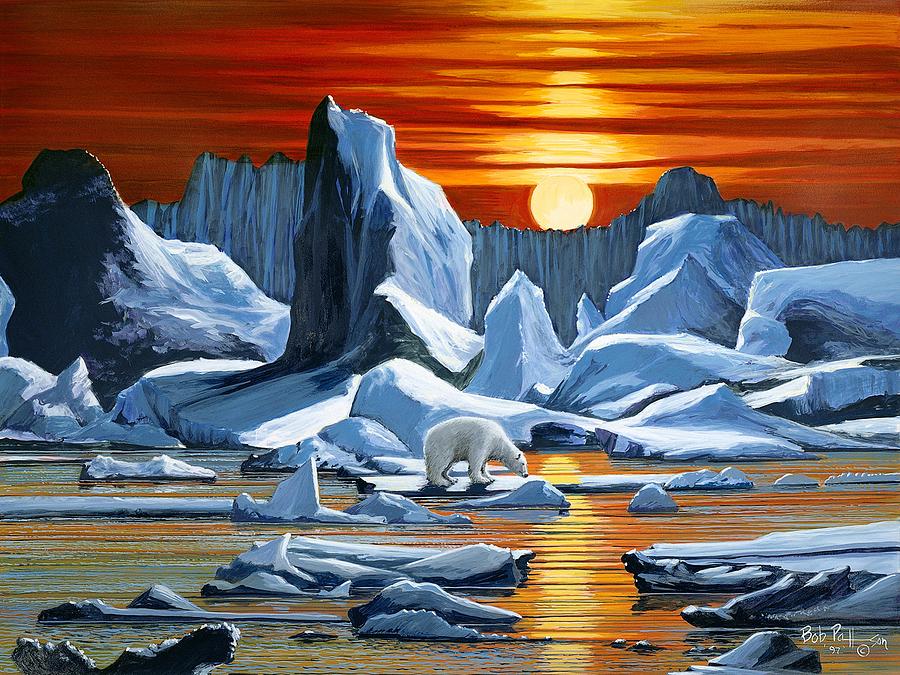The painting features a vivid arctic landscape under an orange-red sky, dominated by the setting sun that reflects off the icy waters below. In the background, the sun descends behind an imposing ice mountain or wall, creating striking contrasts of yellow and darker orange hues in the sky. The water, interspersed with various ice formations, displays a mix of blues and sunlit oranges. A white polar bear, shown in a natural pose sniffing the ground, stands on a small piece of floating ice, adding a touch of life to the serene but cold scene. The rocky, snow-covered formations and fragmented ice pieces lend the painting a textured, almost lifelike quality, enhancing its detailed and atmospheric portrayal of an arctic sunset.